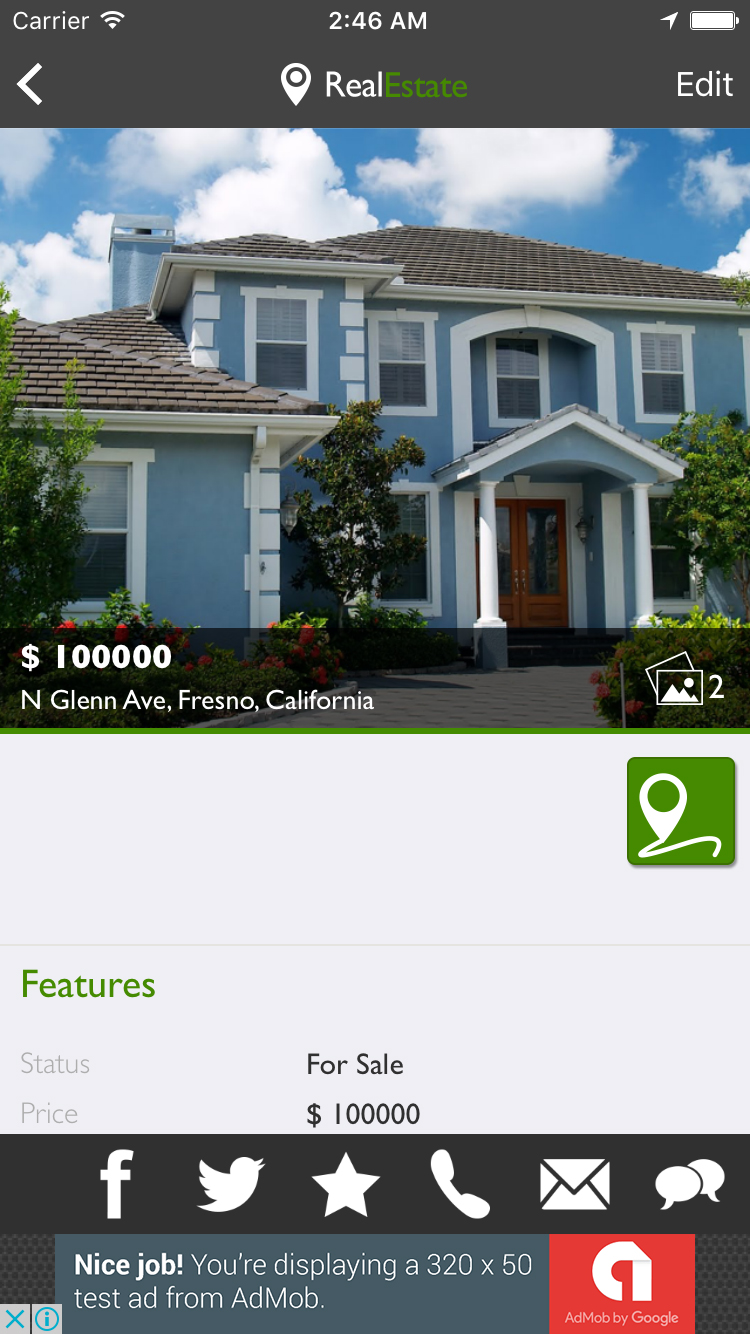A real estate listing page displays a large, two-story house for sale located at North Glen Avenue, Fresno, California, priced at $100,000. The design of the page features the word "Real" in white and "Estate" in green, with a left-pointing arrow and a location pin marking the spot labeled "Real Estate." The top right corner shows service details including the carrier name, Wi-Fi signal strength, the time reading 2:46 a.m., a white paper airplane icon, and a fully charged battery icon. The house itself is painted in a striking blue color with a beautiful roof and distinctive red double front doors. Below the main photo, there is an indication of additional pictures available, labeled "features," and reiterates the "For Sale" status along with the price.